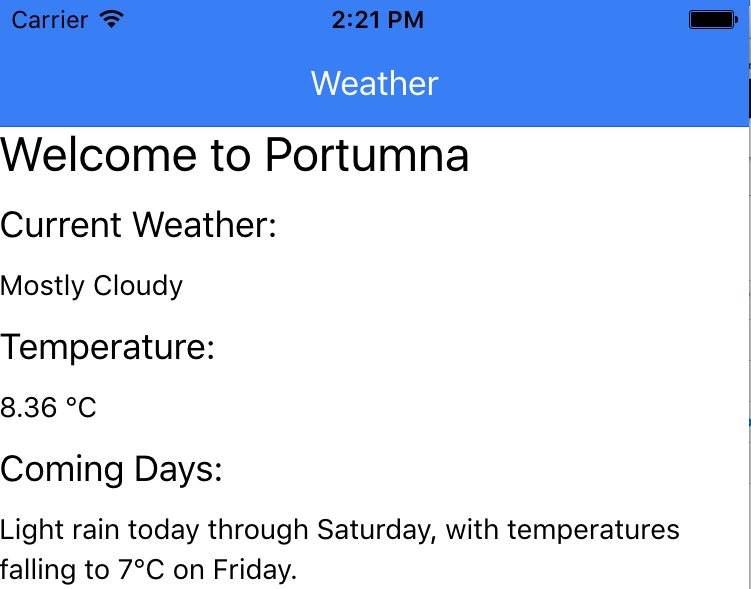The image is a screenshot of a weather report displayed on a smartphone. At the top, the status bar indicates the phone's carrier service, connectivity, the time as 2:21 p.m., and a full battery icon. Below the status bar, within a blue rectangle, the word "weather" is printed in white.

The main section of the screen displays the message "Welcome to Port Umna" in bold and larger black font. Beneath this, the current weather condition is described as "Mostly cloudy." The temperature is listed as 8.36 degrees Celsius.

The forecast for the coming days is summarized with the note: "Light rain today through Saturday with temperatures falling to seven degrees Celsius on Friday." A vertical line runs along the right side of the screen from top to bottom, slightly marking the boundary of the display. 

Additionally, the connectivity status is illustrated with a rainbow-like arc next to the word "carrier" in the status bar.